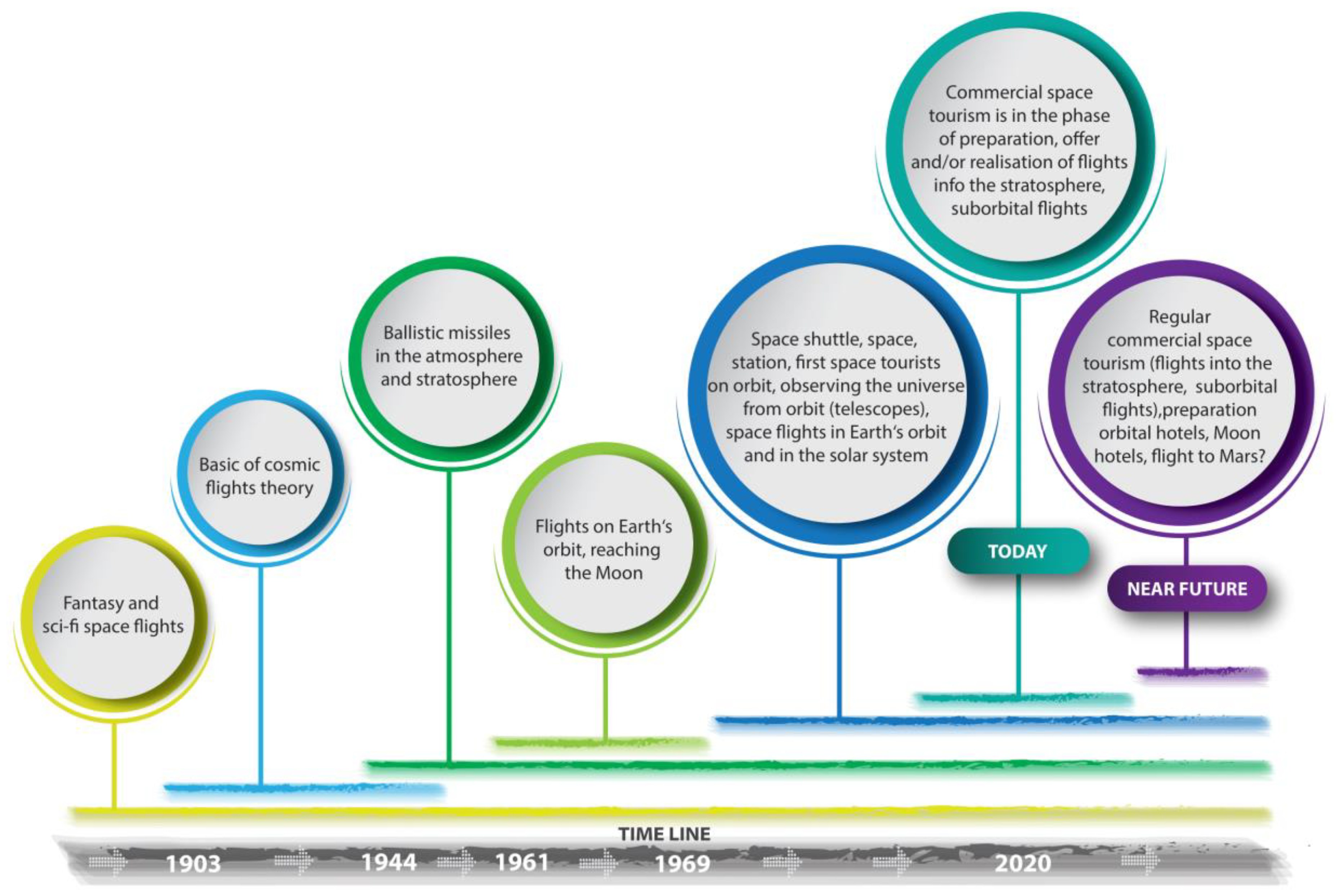The image is a detailed educational slide depicting a timeline that charts the evolution of space flight concepts from fantasy to potential future achievements. At the bottom of the image, a gray bar spans from 1903 to beyond 2020, marking significant years: 1903, 1944, 1961, 1969, and 2020. Above this bar, colored lines and circles map out key milestones.

Starting on the left, a yellow circle marked "Fantasy and Sci-Fi Space Flights" represents the early imaginative concepts of space travel. Moving right, a blue circle labeled "Basics of Cosmic Flight Theory" reflects the foundational scientific principles developed by 1944. A green circle follows, highlighting the era of "Ballistic Missiles in the Atmosphere and Stratosphere."

As the timeline progresses, a lime green circle denotes "Flights on Earth’s Orbit Reaching the Moon," capturing the achievements leading up to the 1969 moon landing. Another significant milestone is represented by a large blue circle, charting the period of "Space Shuttle, Space Station, First Space Tourist on Orbit, Observing the Universe from Orbit, Telescopes, Space Flights in Earth’s Orbit and in the Solar System," which spans developments between 1969 and 2020.

In 2020, a turquoise circle signifies "Commercial Space Tourism in the Phase of Preparation," indicating the nascent state of commercial space endeavors involving stratospheric and suborbital flights. Looking ahead, a purple circle towards the end of the timeline envisions the "Near Future," with "Regular Commercial Space Tourism," featuring suborbital flights, "Orbital Hotels," "Moon Hotels," and the speculative "Flight to Mars."

The timeline cohesively illustrates the progression from speculative ideas to tangible advancements and future possibilities in space travel, color-coded for clarity and structured to highlight the milestones in space exploration and commercial space tourism.